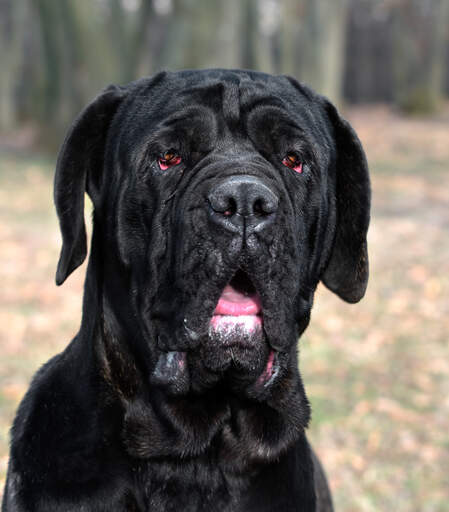This close-up photograph features a large black dog with long, floppy ears and saggy jowls, possibly a mix of a Mastiff or hound breed. The dog has a slightly open mouth, revealing a bit of its lower teeth and tongue. Its eyes are strikingly bloodshot red, almost as if added to the photo, giving it a somewhat sad and weary expression. The black fur appears short and neatly groomed, with noticeable wrinkles around the eyebrows and eye area. The background is entirely out of focus, but it seems to consist of grassy terrain with some leaves and perhaps trees, creating a soft, natural setting that contrasts with the dog's dark figure. Despite the dog's large size and imposing presence, it does not look particularly happy.